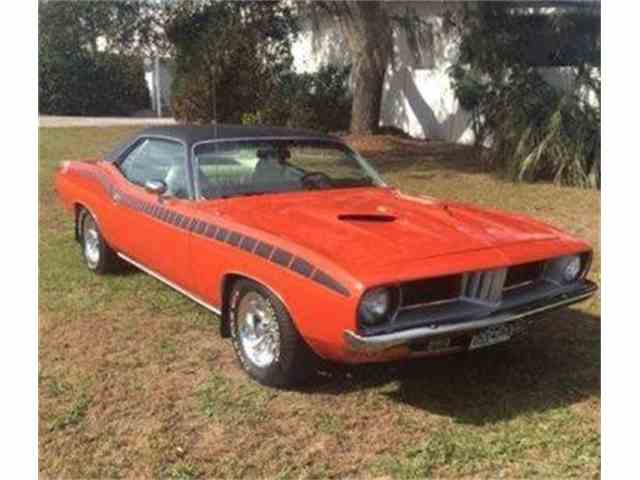The image depicts a vintage orange muscle car, likely from the 1960s, positioned on a mostly dead grass lawn in front of a white house with a white fence and several shrubs. The car, identified as a Lee Barracuda, features a distinctive black roof and a series of black stripes along its side, including a long skinny triangle and a sequence of squares. The car showcases perfect circular headlights and a grille consisting of four small lines, located above a chrome bumper with a white front license plate. Additional details include a visible steering wheel through the windshield. The scene also features a large tree, more bushes, a trimmed hedge, and part of a driveway on the left.